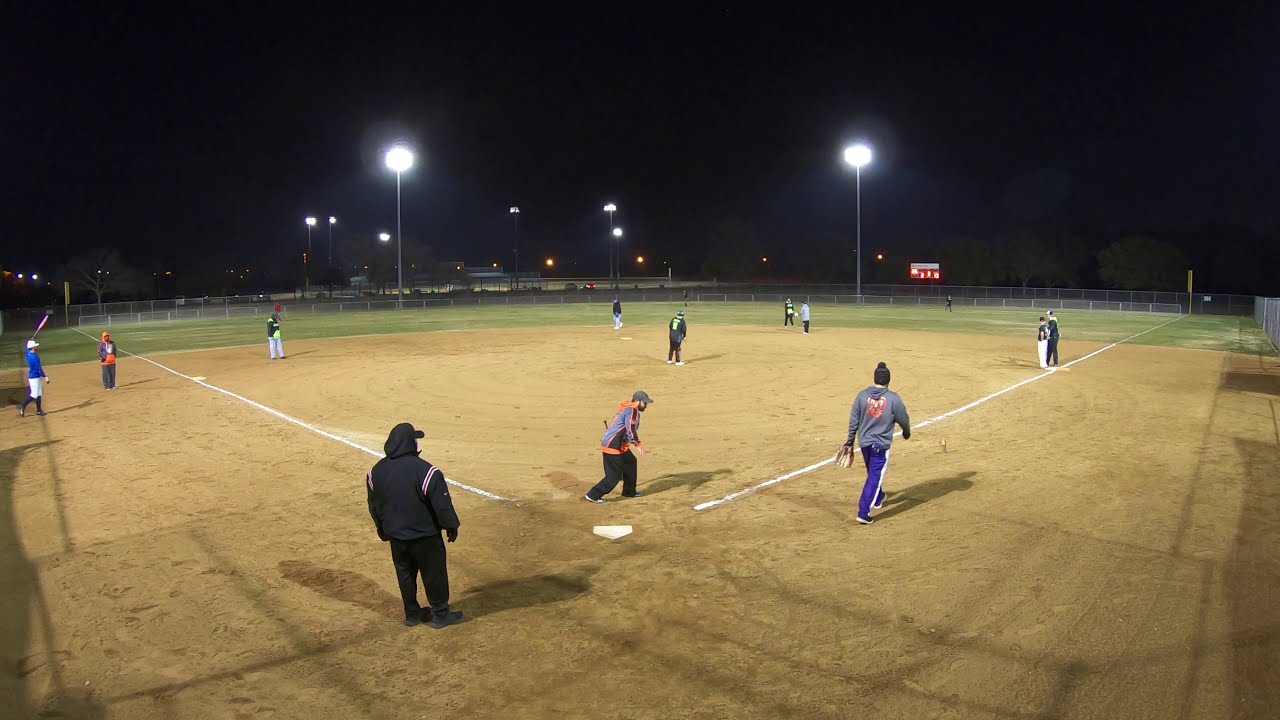The image depicts a nighttime scene at a softball field. The viewpoint is from behind the home plate, looking out over a light brown clay dirt infield area, clearly defined by white outlines marking the bases and a prominent white triangle at home plate. At the front of the image, near the infield corners, stands a man wearing a black coat with a hood over a ball cap, possibly the umpire or an official. Scattered around the field are several players, some casually dressed while others wear gray jerseys with neon yellow accents, suggesting a friendly game among acquaintances.

The green outfield stretches beyond the infield, while the entire field is enclosed by a distant fence. Tall lampposts line the perimeter of the field, illuminating the scene under a dark sky. Additional lights and a scoreboard are visible far in the background, completing the setup of this nighttime baseball game. The descriptive details vividly convey the casual, community-oriented atmosphere of the game, with its mix of informal and slightly more organized elements.